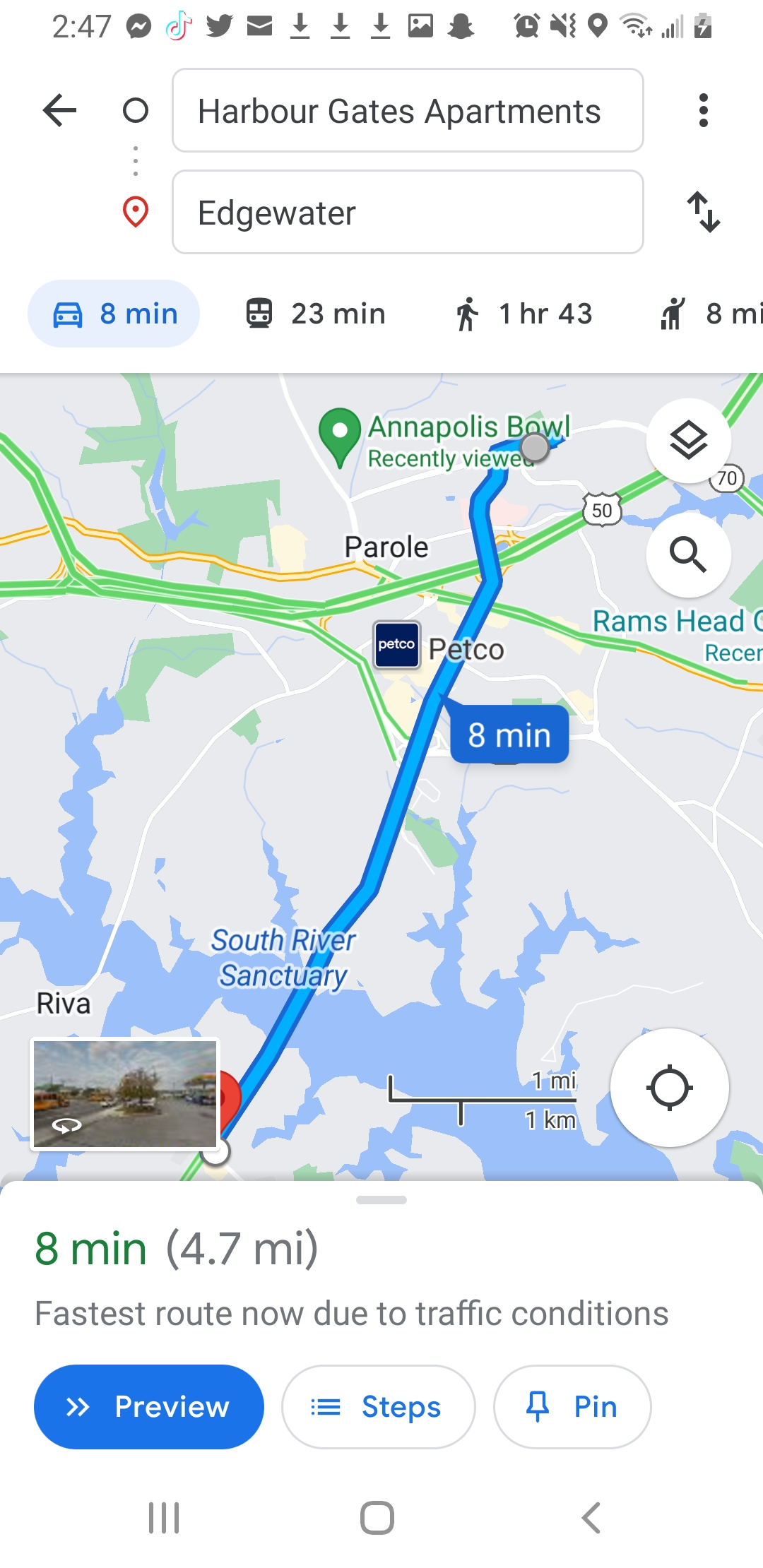This image is a screenshot of Google Maps, depicting a navigation route. The route, displayed in various map symbols and icons familiar to mobile users, begins at "Harbor Gates Apartments" located prominently at the top left. The interface shows standard mobile elements such as a signal bar, battery meter (with half charge), and a row of app icons, including SMS, TikTok, Twitter, Email, three download symbols, an image icon, and a Snapchat symbol. An alarm call and location symbol are also visible. The navigational path extends 4.7 miles to Annapolis Mall, requiring approximately 8 minutes of travel. The route traces a northward direction from Harbor Gates Apartments, crossing a river. Green text at the bottom of the image confirms the estimated travel time as 8 minutes, contingent on current traffic conditions.